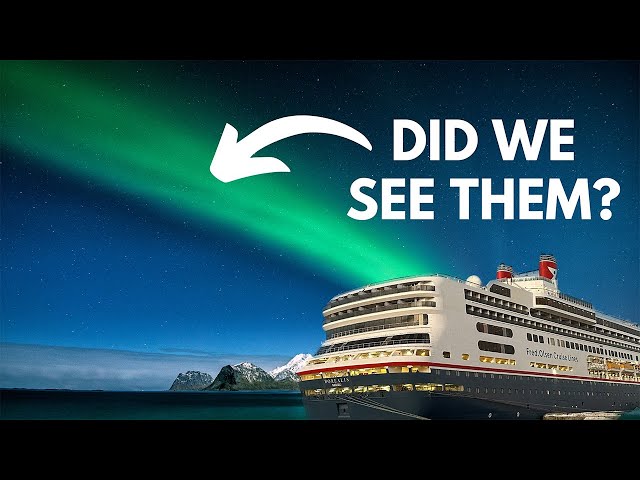This image, likely a YouTube thumbnail or an ad poster, vividly captures the magical experience of viewing the Aurora Borealis from a cruise ship. Dominating the scene is a large white cruise ship with a dark gray bottom and numerous windows, featuring red funnels and a stripe. The ship, branded with the text "First Class Cruise Lines," is sailing from the right to the left against a backdrop of a dark sea, distant snow-capped rocks, and hills. Above, the night sky transitions from deep blue to dark with twinkling stars and neat clouds extending leftward. A stunning display of the Northern Lights, in vivid green, stretches from the upper left corner down to the ship. Adding to the allure, a prominent white arrow points to the Aurora Borealis with the text "Did we see them?" set in block letters, highlighting the ethereal spectacle. The composition's striking yet straightforward color palette enhances the enchanting scene, inviting viewers to share in the awe of this natural wonder.